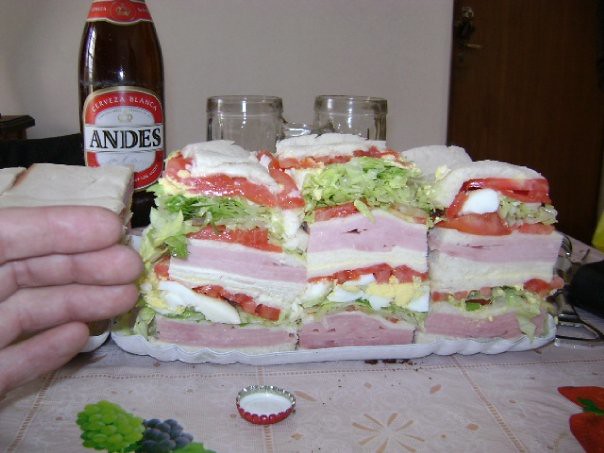In this photo, there's a detailed scene of a kitchen table adorned with a vibrant pink tablecloth with patterns of grapes, strawberries, and blueberries. Central to the image is a white plate piled high with dense, towering sandwiches. The sandwiches are stacked with layers of pink ham, thick tomato slices, shredded lettuce, melted cheese, and boiled eggs, all alternating in a visually chaotic manner. To the left, four light-complexioned fingers seem to present the sandwiches proudly. In the background, a brown bottle of Andes beer prominently features a red and gold label and sits beside two inverted crystal-clear mugs. An upside-down red bottle cap, likely from the beer, rests beside the sandwiches. The backdrop includes a white wall and a wooden piece leaning against it, adding to the casual kitchen ambiance. Overall, the image is a vivid, cluttered depiction of an informal yet hearty meal setup.